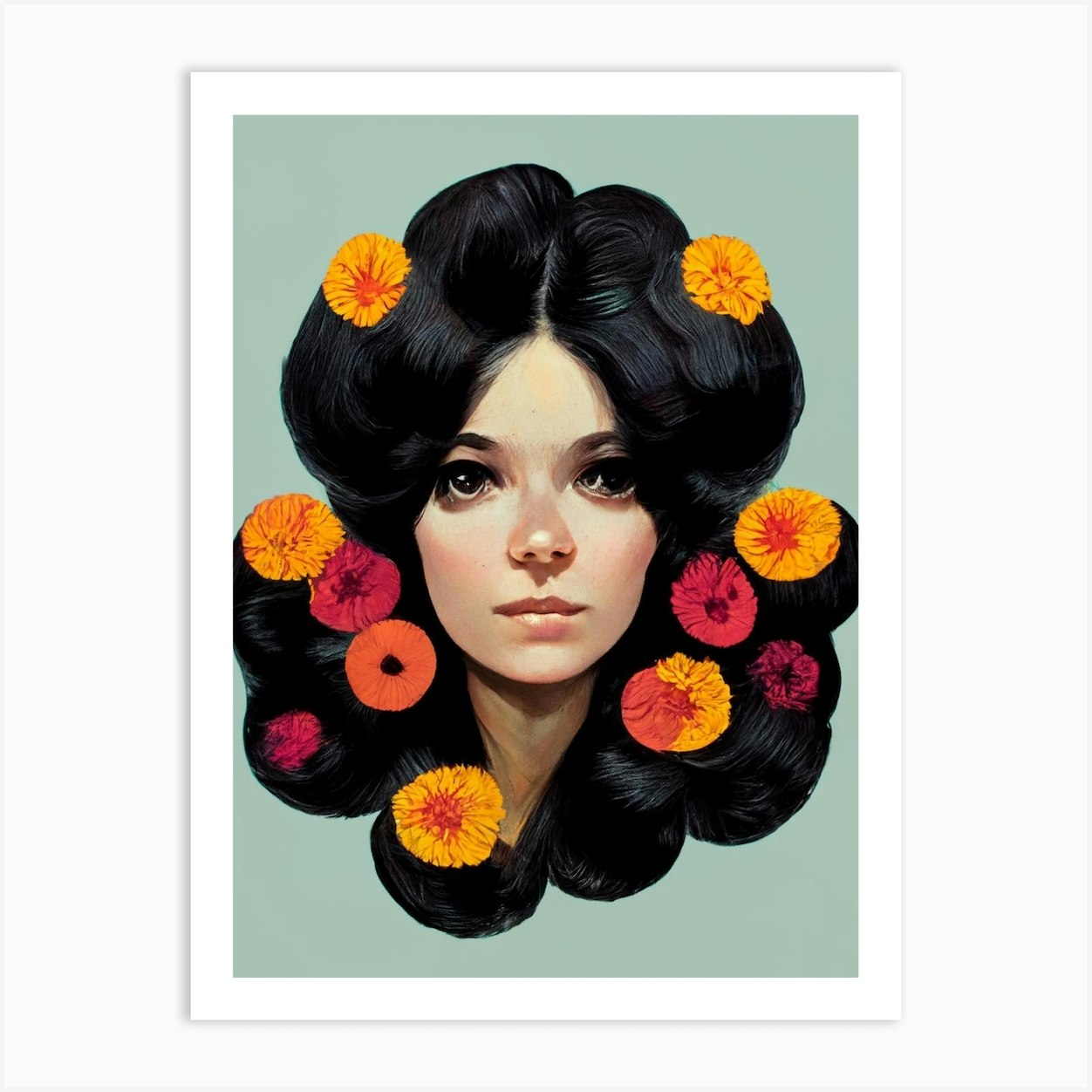A vertical rectangular painting hangs on a pure light gray wall, encased in a subtle gray shadow. The artwork features a sand green matte background and depicts a woman's head with large, dark eyes and neatly manicured, voluminous black hair. Her hair is styled in an intricate array of curls and buns, cascading around her face and shoulders. Adorning her hair is an assortment of vibrant flowers: Five bright orange flowers are positioned symmetrically—two at the top, two on each side, and one at the bottom. Four reddish-pink flowers form an arc across the center, accompanied by a deep orange bloom beneath the leftmost pinkish-red flower. At the bottom right, a half-and-half yellow and red flower is nestled within the hair. The flowers vary in shades from dark orange to light yellowy orange and resemble various types of chrysanthemums and daisies. The painting's white border frames the detailed and lifelike portrayal, emphasizing the elaborate floral arrangement and the woman's serene expression.